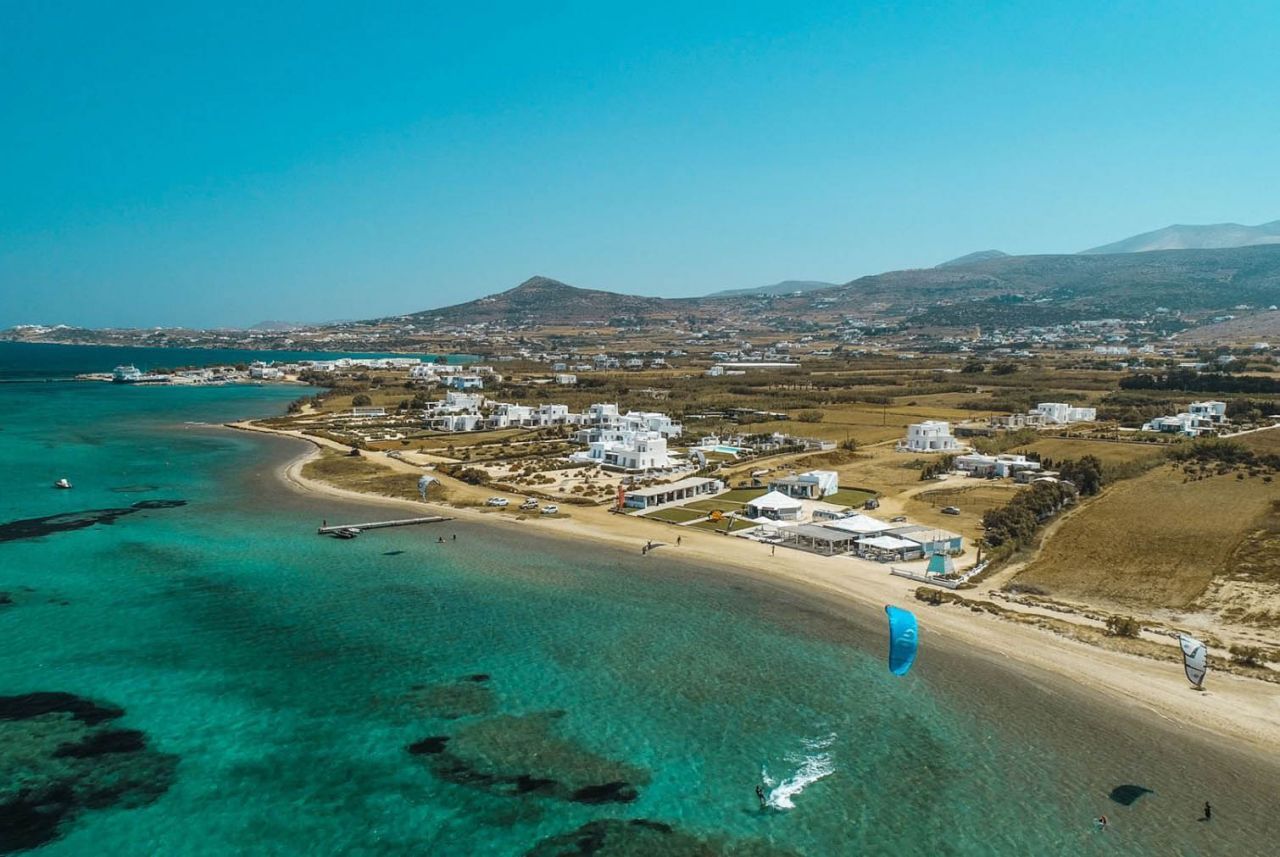This scenic aerial view presents a tranquil coastal town, centered with its characteristic cluster of mostly white buildings, giving a charming and serene atmosphere. The beach stretches along the coastline, transitioning from dull olive-green grass to sandy shores that meet the ocean's edge. The ocean itself shifts gradually from a light aqua near the shore to a deeper blue further out. The left and bottom parts of the image are dominated by the ocean, where rocks are visible beneath the surface, and a dock extends out with a small boat moored to it. Nearby, a windsurfer with a distinctive blue sail glides through the water, while a few people enjoy the beach and water. Cars are parked along the shoreline, and metal canopies add to the infrastructure visible in the scene. In the background, a series of hills and mountains rise, sprinkled with additional buildings and sparse vegetation, creating a layered, picturesque landscape under a clear, sunny sky.